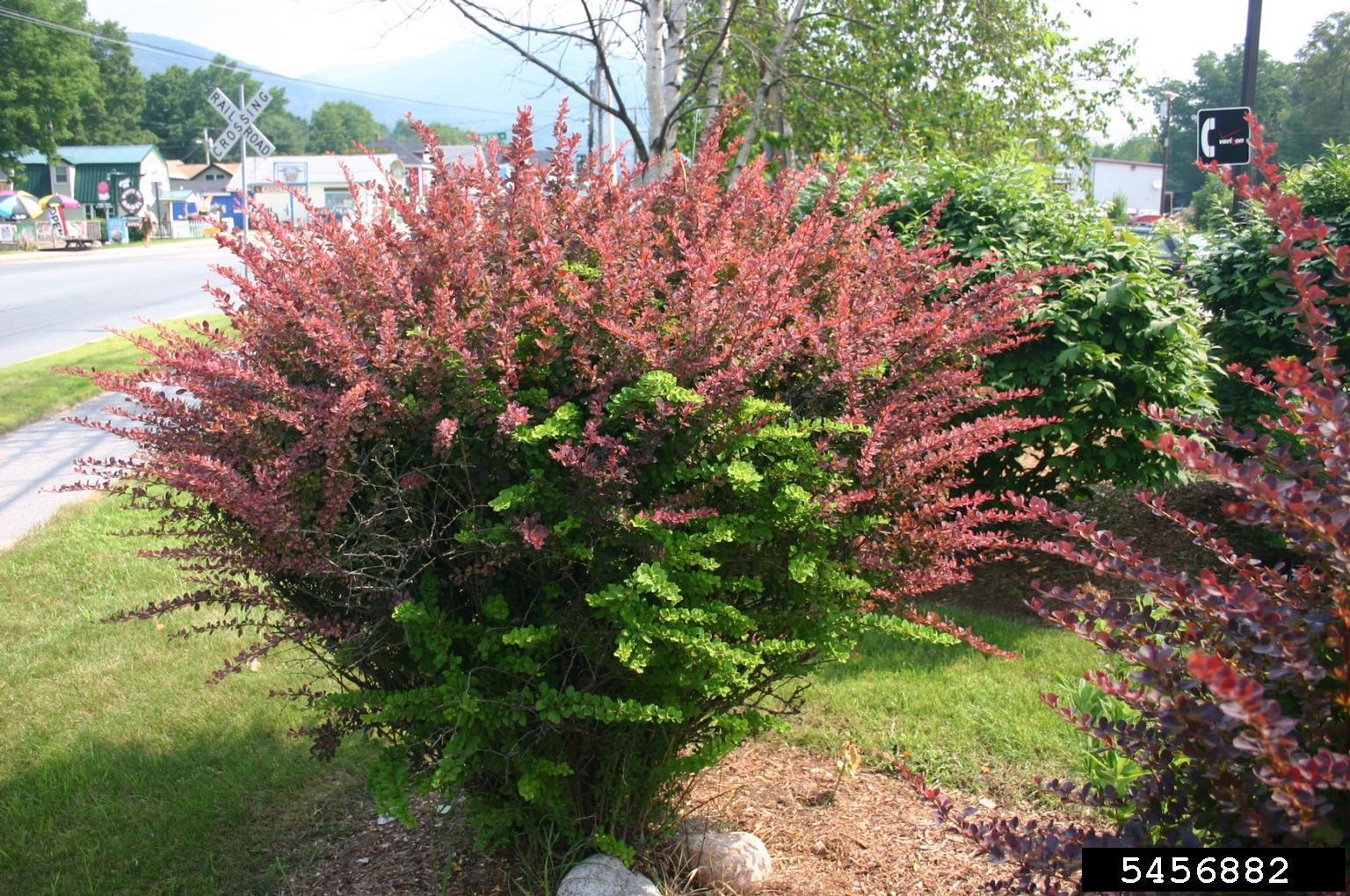In this outdoor daytime photograph, we see a bush with green foliage at its base and tall, red stems extending upwards, forming a cone-like shape. The bush is situated in a grassy area adjacent to a sidewalk that runs along the left side of the image. A secondary bush with similar features is partially visible on the right edge of the photo. Behind the bushes, there are more shrubs and trees, providing a lush backdrop. A black banner with white numbering, "5456882," is located at the bottom-left corner of the image.

In the midground, we see a street lined with small buildings, resembling a quaint small town. A distinct railroad crossing sign is positioned just beyond the bush on the same side of the road. Further into the background, a telephone pole with a "Verizon" sign featuring a small white phone icon is visible among additional trees, contrasting against the white sky seen in the upper portions of the image.